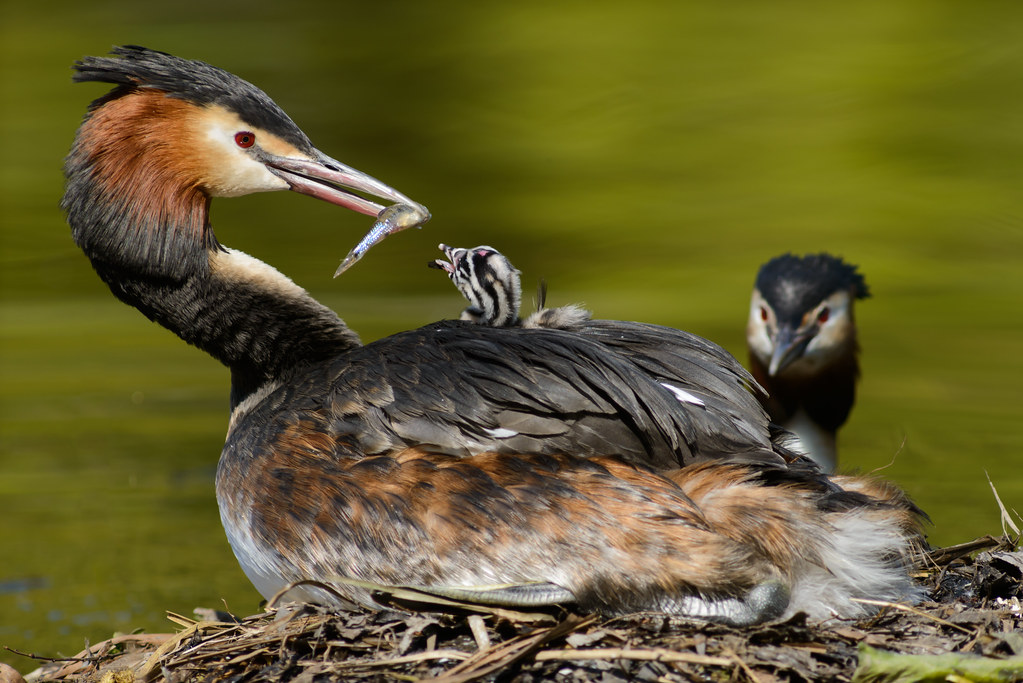This is a horizontally-aligned rectangular photograph depicting a tender moment between a mother duck and her baby, with another adult duck observing in the background. The scene is set in an outdoor nesting area composed of light brown twigs and grasses in the foreground. The mother duck, showcasing a mix of dark brown, reddish-brown, black, and gray feathers, is positioned in the center with her body facing away from the camera. Her head is turned around to the right, revealing a long red beak and a distinctive black streak running down her otherwise dark head. The mother duck holds a small silver fish in her beak, ready to feed her baby.

The baby duck, perched on the mother's back, eagerly stretches its neck upwards with its mouth wide open, displaying a striking pattern of black and white stripes on its head, reminiscent of a zebra. In the blurred green background, the faint outline of another adult duck is visible. This duck has a black head with lighter patches around its eyes and beak, and it appears to be observing the feeding interaction.

Overall, the combination of the mother's detailed feather patterns, the baby's striking head stripes, and the serene, blurry green backdrop creates a vivid and touching portrayal of nurturing in nature.